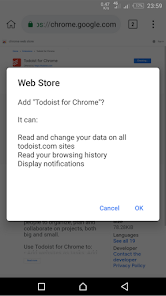This image is a screenshot taken from a phone, capturing a notification from the Chrome Web Store app. The background of the image is grayed out, emphasizing the notification which occupies approximately 50% of the screen's center. The notification features a prominent white rectangular shape that stands out sharply against the dimmed backdrop. 

On the left side of this notification, the bold black text reads "Web Store." Just below, a smaller, dark gray text asks, "Add 'Todoist for Chrome'?" indicating a request for permission to install the "Todoist" app on the browser. The notification details the permissions required by the app, stating: "It can read and change your data on all todoist.com sites, read your browsing history, and also display notifications." 

At the bottom of the notification are two actionable buttons, "Cancel" and "OK," both presented in a mid-blue color. The backdrop hints that the browser in use is Chrome, visible from part of the URL bar at the top, which reads "chrome.google.com". This URL bar further confirms that the screenshot was taken while navigating the Chrome Web Store.